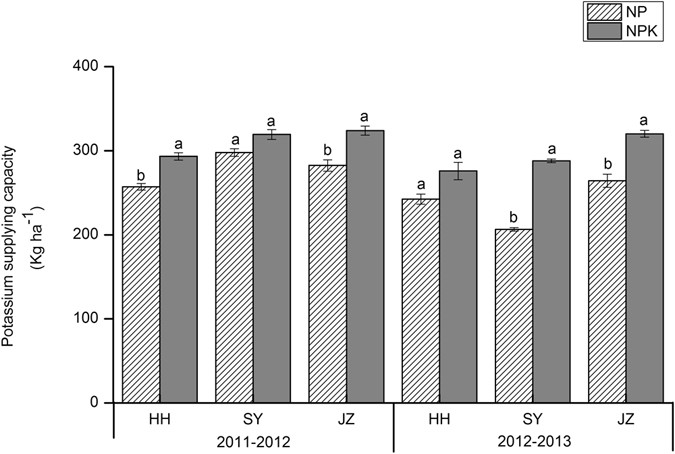The black and white bar graph illustrates the potassium supply capacity measured in KG HA⁻¹. The y-axis scales from 0 to 400, incrementing by 100, while the x-axis is segmented into two primary groupings representing the periods 2011-2012 and 2012-2013. Each primary grouping is further divided into four sub-segments labeled HHSYJZ. Each segment includes two bars: NP, shaded with diagonal stripes, and NPK, shaded solid gray. Across all groupings and years, NP and NPK appear side by side, with NP generally lower than NPK. The data suggests a slight year-over-year decrease in potassium supply capacity for both NP and NPK, though overall levels remain consistent within each time frame. Specifics show the relative measurements and groupings HHSYJZ, indicating differences in potassium supply across these segments, although the significance of these particular segment labels (HHSYJZ) remains unclear without further context.